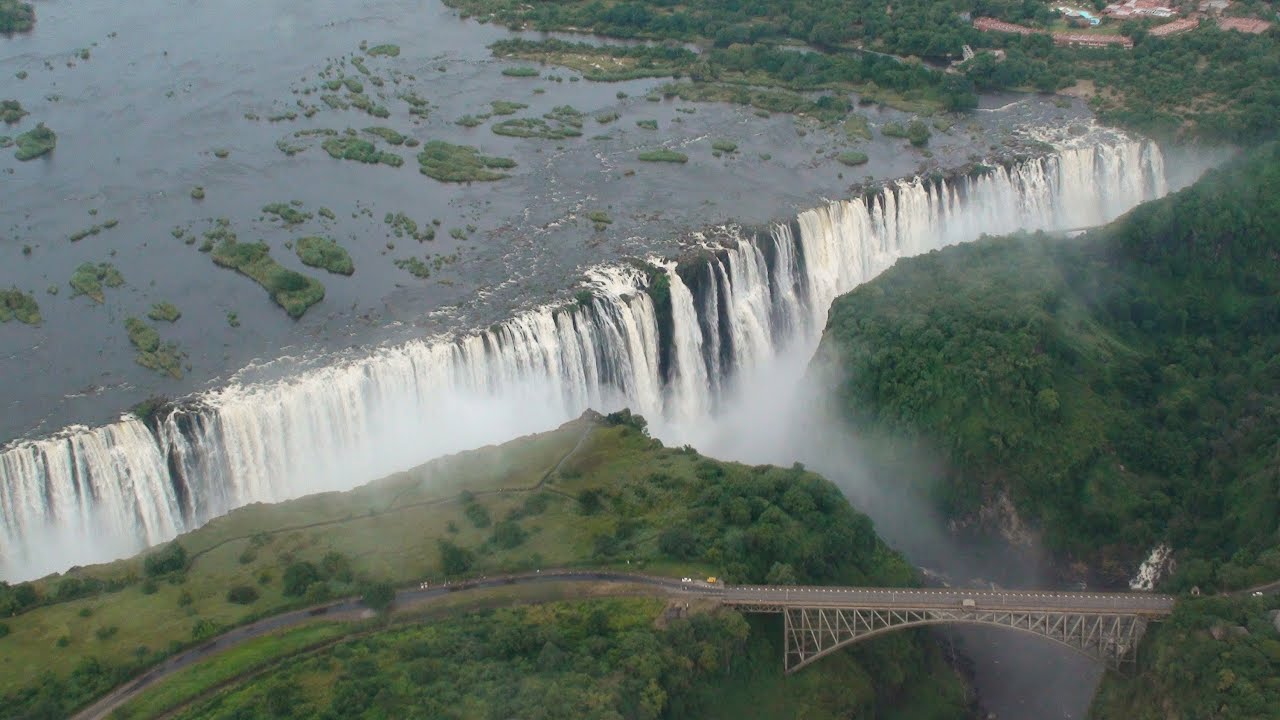This aerial photograph captures the stunning landscape of a massive, broad waterfall plunging into a narrower river flanked by dense forested areas. The waterfall spans nearly the entire width of the image, characterized by segments of break and rocks at its crest. Mist rises from the powerful descent, adding a hazy atmosphere to the scene. In the background, faintly visible are some red-roofed buildings set against a stretch of land, indicating a distant human presence. Above the falls, the river is dotted with clumps of greenery and small islands, suggesting shallow depths at parts. From the upper left corner, a two-lane road meanders across the image, curving to the right and crossing over a high trestle bridge that spans the narrow waterway created by the waterfall. This bridge, which accommodates visible car traffic, connects the two lush forested areas in the foreground. Overall, the image showcases a vibrant mix of natural splendor and slight human development, encapsulated in the grandeur of the waterfall and its surrounding landscape.